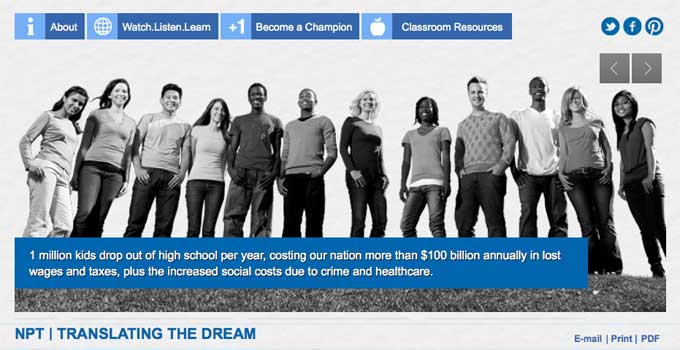This black-and-white screenshot showcases a landing page for NPT (National Public Television), highlighting their educational initiative called “Translating the Dream: Watch, Listen, Learn, Become a Champion.” The upper section of the image is characterized by a blue navigation bar with white text, while the remainder of the image remains in shades of gray, black, and white.

The central visual element is a collage of people standing in a field, rendered in a grayscale palette. In the middle of this monochromatic composition, a significant statistic is displayed in bold text: "1 million kids drop out of school per year, costing our nation $100 billion annually in lost wages, taxes, plus the increased social cost due to crime and healthcare."

Social media icons for Facebook, Twitter, and Pinterest are displayed beneath the statistic, along with options to email, print, or download the information as a PDF, all outlined in a blue banner at the bottom of the image. The overall effect is a stark, impactful presentation that underscores the gravity of the educational challenges faced by the nation.

The screenshot captures the essence of NPT’s mission, offering educational resources to help mitigate the dropout crisis and foster champions in the classroom.